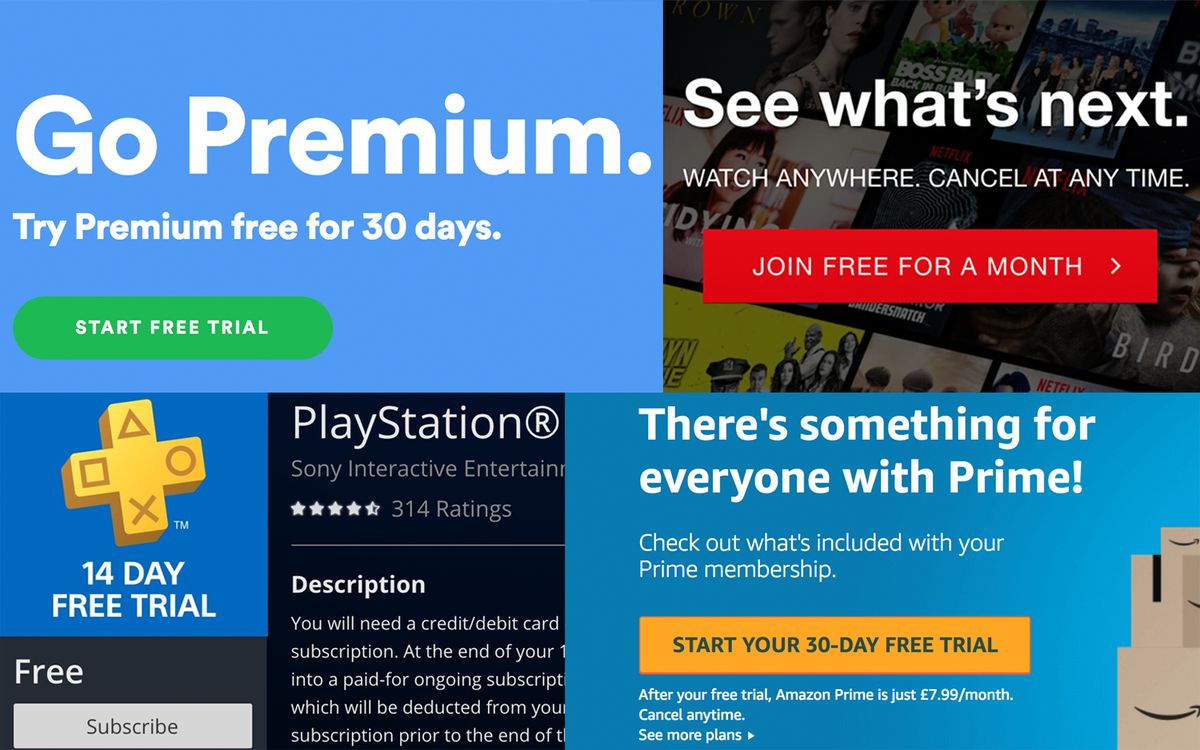The image appears to be a promotional page from Sony Interactive Entertainment. The page is approximately seven inches wide and five inches tall, divided into various sections. 

In the top left, there is a call to action with a prominent message: "Go Premium - Try Premium Free for 30 Days," accompanied by a "Start Free Trial" button. 

To the right of this section, there's another segment inviting users to "See What's Next," "Watch Anywhere," and "Cancel at Any Time," along with another prompt to "Join Free for a Month." This area features images of television series and movies, indicating some type of streaming entertainment service.

On the bottom left, there's an image of a game controller icon within a square, showcasing directional buttons (left, right, up, down). It promotes a "14-Day Free Trial" and encourages users to "Subscribe for Free." Adjacent to this, additional details about PlayStation and Sony Interactive Entertainment are displayed, including a rating of 4.5 stars based on 314 reviews. It notes that a credit card is required, and subscription fees will be automatically deducted at the end of the free period.

In the lower right, another section highlights "Something for Everyone with Prime," urging users to check out what is included with a membership. It prompts visitors to "Start Your 30-Day Free Trial," although it’s unclear whether this refers to Amazon Prime or a similar service provided by Sony Interactive Entertainment.